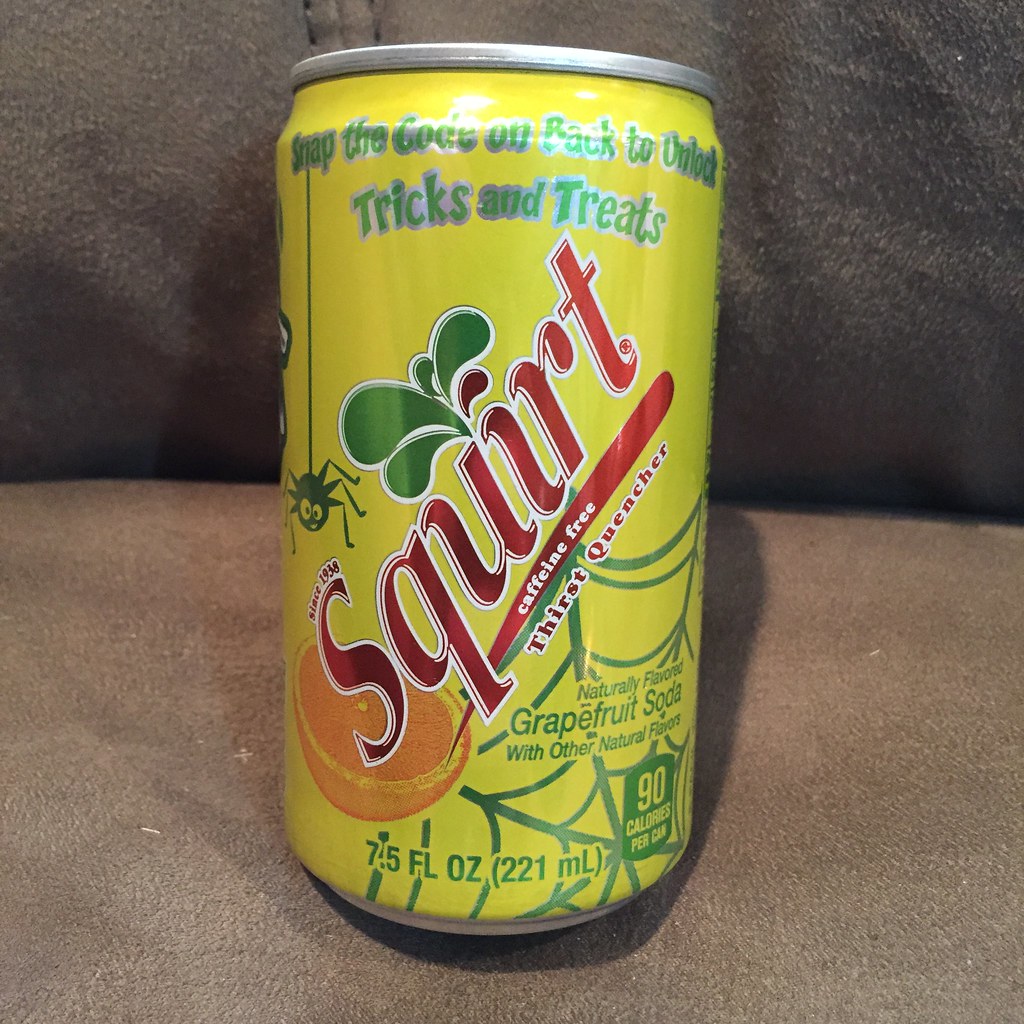The photograph features a 7.5 fluid ounce (221 milliliters) can of Squirt soda prominently positioned on a sturdy brown chair, which appears to be made of leather or possibly vinyl material. The chair's seat is a lighter brown while the backrest is darker, and visible stitching details can be observed in the top left corner near where the can rests against it. The can itself is primarily yellow and green, with the Squirt logo written in vibrant ruby red and adorned with a graphic of a grapefruit slice suggesting its grapefruit soda flavor. The can bears festive Halloween-themed decorations, including a spider hanging down from the word "snap" at the top, part of the text "snap the code on the back to unlock tricks and treats." Additional text declares it to be "caffeine-free thirst quencher" and "naturally flavored grapefruit soda with other natural flavors." The can, compact and distinctive, stands out against the background of the chair, merging both mundane and festive elements in a single, detailed scene.